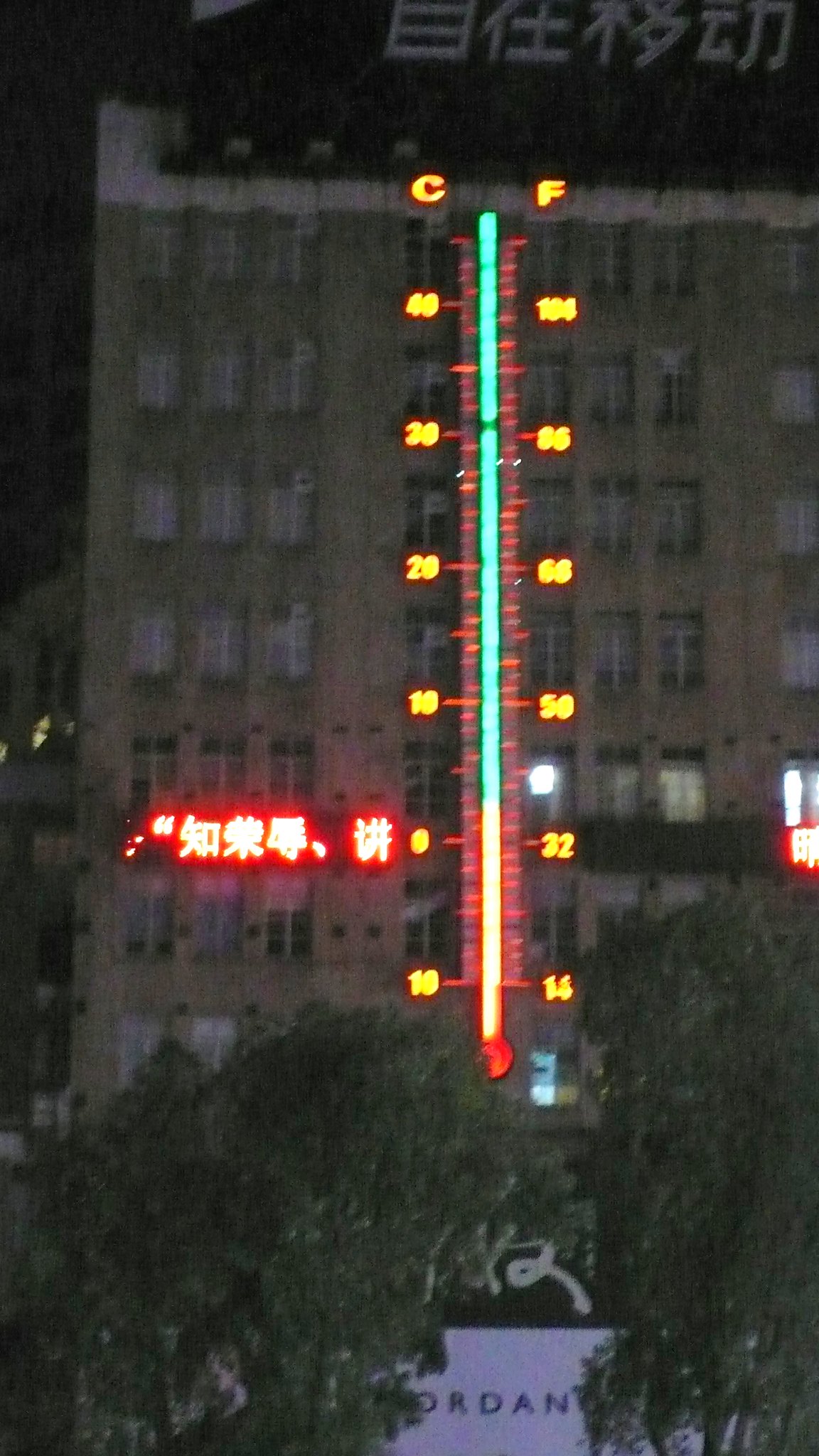The image depicts the facade of a tall, eight-story concrete building with a gray exterior and white-framed windows, captured during nighttime. A striking feature of the building is a giant wall thermometer that stretches vertically from the first floor to the rooftop. This thermometer, illuminated in vibrant LED lights, showcases a red bulb at the bottom, transitioning through yellow and green lights as it climbs upward. The left side of the thermometer is marked with a "C" in yellow LED lights, indicating degrees Celsius, while the right side is labeled with an "F" in the same yellow lights, representing degrees Fahrenheit.